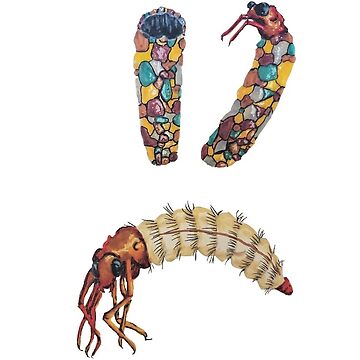The image is a composite illustration depicting the life cycle of a peculiar, shrimp-like insect emerging from a bright, multi-colored cocoon. 

At the top, the image showcases two vibrant, rock-like cocoons, reminiscent of river pebbles, with intricate etchings in shades of blue, yellow, pink, red, and green. These structures appear to be jeweled and thimble-shaped, with open tops resembling black apertures. The leftmost cocoon is empty, while from the rightmost cocoon, an insect with large, black prawn-like eyes and pink appendages is emerging.

Below these cocoons, the insect is shown fully emerged, displaying a red ochre torso with a white, segmented, caterpillar-like tail. The body is adorned with scattered brown hairs and distinct pink lines running along its abdomen. The overall composition vividly illustrates the transformation of the insect, highlighting its transition from the colorful, protective cocoon to its final form with detailed anatomical features.